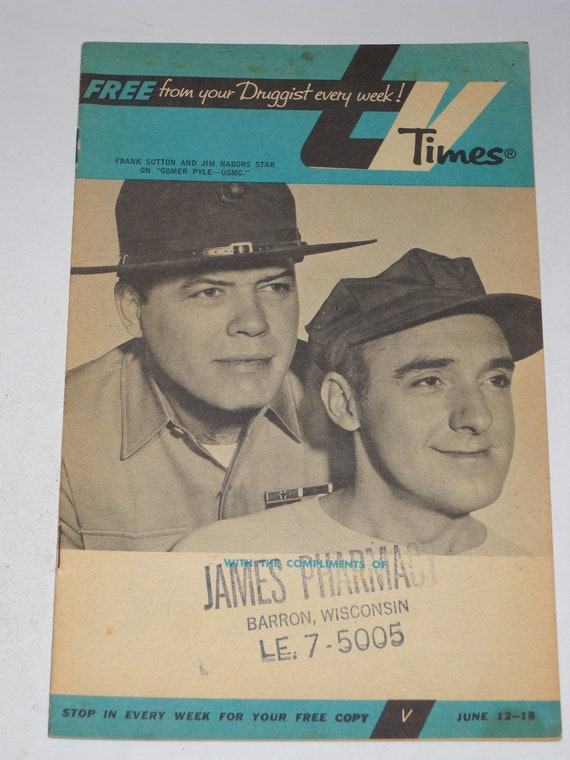The cover of this old TV Times pamphlet, available for free from your local druggist, features a light turquoise banner at the top with retro-style text. It prominently advertises Frank Sutton and Jim Nabors starring in "Gomer Pyle, USMC." Below this banner is a black-and-white photograph of two men in military uniforms; the man in the stern-looking sergeant's hat stands behind the man in a floppy hat with a goofy expression. A rubber stamp imprint on the bottom right corner reads "James Pharmacy, Barron, Wisconsin, LE7-505." The pamphlet encourages readers to "Stop in every week for your free copy," highlighting this specific issue dated June 12th through the 18th. The design is simple and plain, with a nostalgic feel reflected in its monochromatic photo and blue accents.